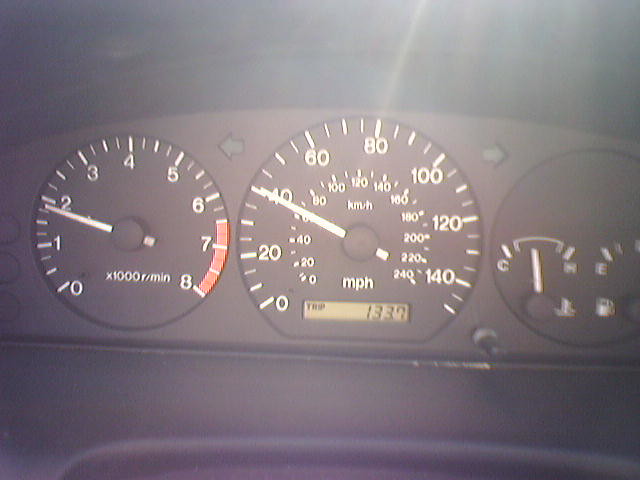This photograph captures the various readouts of a car's dashboard, presumably while the vehicle is in motion. Taken from inside the car, the image showcases the dashboard against a backdrop of a black interior. Central to the composition is the speedometer, which indicates the car is traveling at approximately 41 or 42 miles per hour; this is marked by a white pointer just above the 40 mph mark, with the digital odometer below showing a distance of 133.7 miles traveled.

To the left of the speedometer is the tachometer, which measures the engine's rotations per minute (RPM). The tachometer's white, pointed needle rests just below the 2000 RPM mark, reflecting the engine's moderate activity. On the right side of the speedometer are two additional gauges: an engine temperature indicator on the left half, showing the engine's temperature status, and a fuel gauge on the right, which, although partly cut off in the picture, appears to lean towards the "full" side.

The image has a slightly washed-out look due to the daylight filtering in from the top, casting noticeable sun rays across the dashboard. Despite the glare, the details of the car's controls and readouts remain clearly visible.